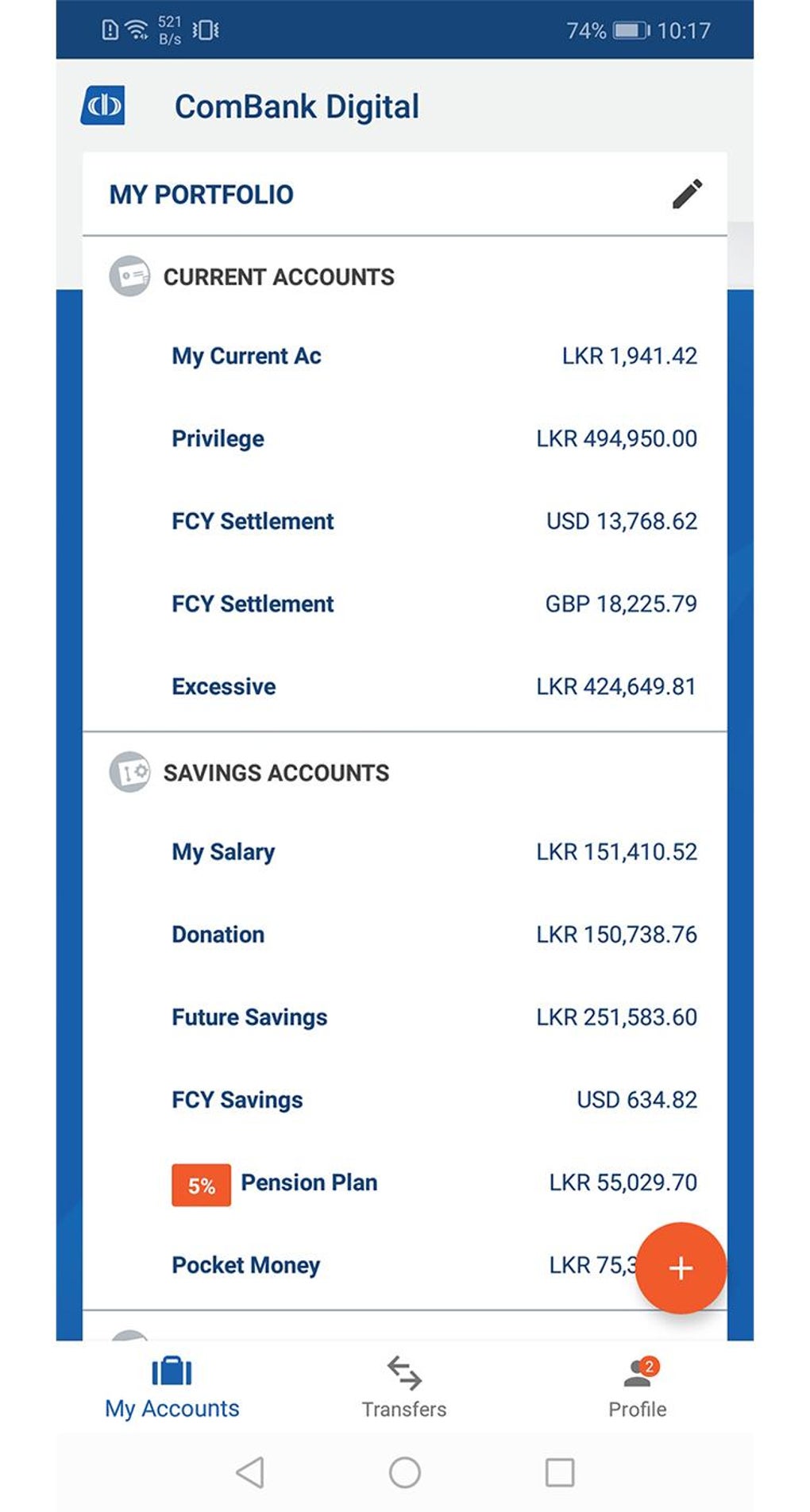This image is a portrait-oriented screenshot displaying a banking app interface. In the upper right-hand corner, the battery level is shown at 74%, and the time is 10:17 AM, all within a blue status bar. Below that, in a gray stripe, the header reads "COMBANK Digital."

The main section features a pop-up menu titled "My Portfolio." To the right of this title is an icon indicating that the user can edit this section. The portfolio is divided into various account categories with their respective balances.

**Current Accounts:**
- My Current AC: LKR 1,941.42
- Privilege: LKR 494,950.00
- FCY Settlement (US Dollars): $13,768.00
- FCY Settlement (Great Britain Pounds): £18,225.00
- Excessive: LKR 424,649.00

**Savings Accounts:**
- My Salary: LKR 151,410.00
- Donation: LKR 150,738.00
- Future Savings: LKR 251,583.00
- FCY Savings (US Dollars): $634.82
- 5% Pension Plan: LKR 55,029.70
- Pocket Money: LKR 75,000.00

At the bottom right-hand corner of the screen, an orange button with a plus sign is present, indicating an option to add more entries or accounts.